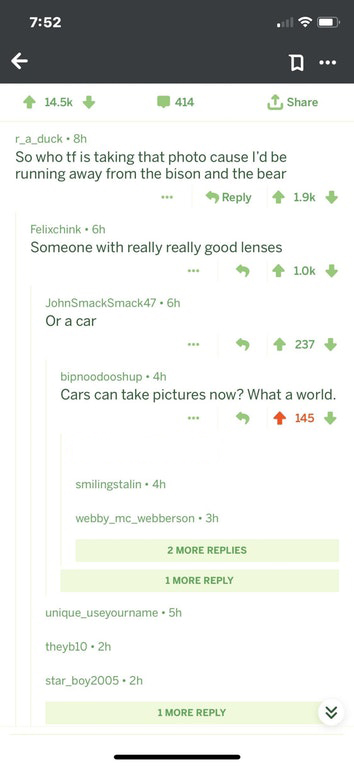A screenshot of a social media post showing a humorous conversation between users reacting to a daunting situation. The top section of the image shows a message exchange where one user says, "So who the fuck is taking that photo? Because I'd be running away from the bison and the bear," suggesting the presence of both wild animals in the photograph. Another user humorously responds, speculating that it must have been taken by "Someone with really, really good lenses or a car. Cars can take pictures now. What a world."

The post, striking a chord with many, has amassed significant engagement with 14.5K likes. The conversation continues with additional replies over time: two more responses eight hours ago gaining 1.9K likes, one reply six hours ago getting 1,000 likes and another six hours ago with 237 likes. A later comment made four hours ago has 145 likes.

Users involved in the conversation include:
- Starboy, 2005
- They be tan
- Unique username
- Webby McWeberson
- Smiling Stalin
- Bip noodle soup
- John smack smack, 47
- Felix chinks are a duck

The bottom of the image shows that the content is captioned: "Subs by www.zeoranger.co.uk," indicating the source of the subtitles or transcriptions.